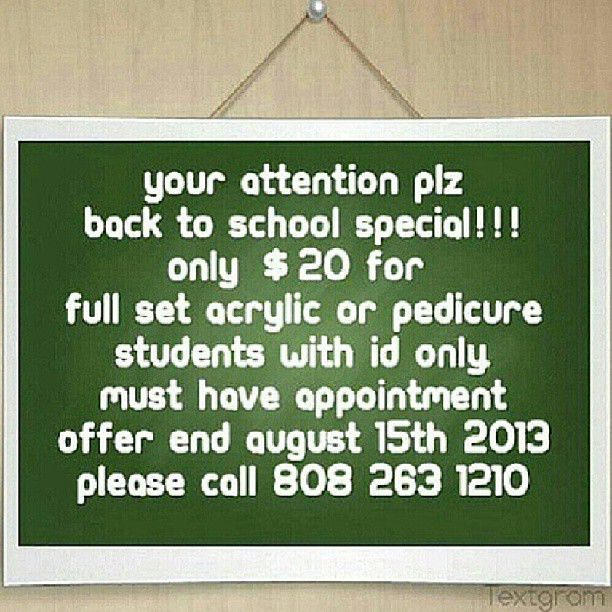The image depicts a sign hanging on a light-colored, paneled wall, secured by a string that creates a triangular shape fastened to a metal hook at the top. The sign consists of a white border with a dark green background. The message is written in small, white letters and is formatted as follows: 

"Your Attention PLZ. Back to School Special!!! Only $20 for Full Set Acrylic or Pedicure. Students with ID Only. Must Have Appointment. Offer End August 15th, 2013. Please Call 808-263-1210."

In the bottom right corner, there is a digital watermark reading "Textgram." The sign, intended for students, emphasizes the necessity of an appointment and includes a phone number for scheduling. The overall presentation lacks the name of the establishment and features informal grammar and spelling.